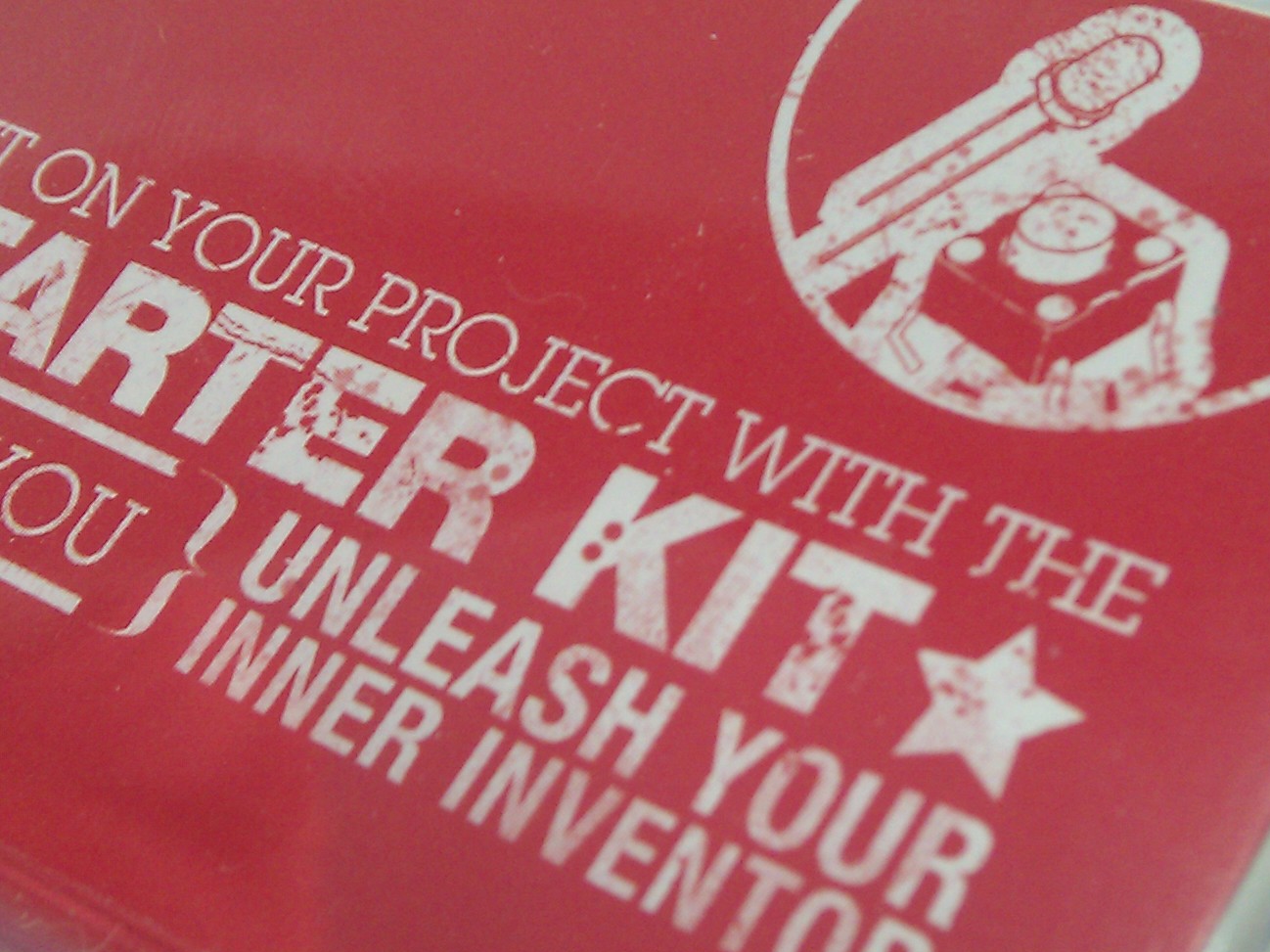The image features a red background with partially visible white text. The text appears fragmented, capturing only the lower halves of the letters. At the top right corner, there's an icon resembling either a stop button or a switch, also in white with a red outline. The visible text reads: "On your project with the starter kit" and is accompanied by a white star icon. Below this, the partially obscured phrase, "Unleash your inner inventor," is visible, though the letter "R" in "inventor" is cut off. The overall appearance suggests the text is intentionally faded, likely a stylistic choice. Additionally, components of an LED and a switch with legs that connect to a motherboard are seen at the top right, enhancing the tech imagery consistent with a starter kit theme.